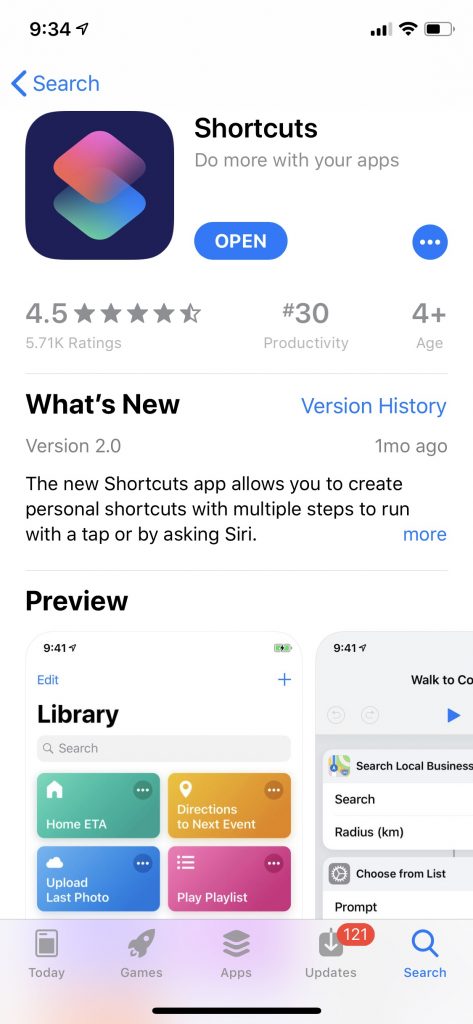This screenshot captures a detailed view of an app store page for the Shortcuts app. At the top, the status bar shows the time as 9:34 AM, a paper airplane icon indicating airplane mode, a Wi-Fi symbol, signal strength indicator, and a battery icon. Below the status bar, there's a search bar with the word "search" in blue text.

Immediately below, a navy blue box features pink and teal icons and text in black reading, "Shortcuts: Do more with your apps." Adjacent to this description is a blue and white box labeled "Open" and a blue and white circle with three dots.

Scrolling down, the app has a rating of 4.5 stars based on 5.71K ratings, is ranked number 30 in productivity, and is indicated to be suitable for ages 4 and up. The section titled "What's New" mentions version history in blue and black text, with the latest version 2.0 released one month ago. This update allows users to create personal shortcuts with multiple steps to execute commands via tap or by asking Siri, with a "more" button in blue for additional details.

The "Preview" section details mini screenshots of the app interface: one screenshot shows tabs labeled "Edit," "Library," and "Search," with four colored boxes below. The teal box reads "Home ETA" with a home icon, the orange box shows location pins and "Directions to next event," the blue box has a cloud icon with "Upload last photo," and the pink box displays a list icon with "Play playlist."

A secondary screenshot on the side indicates the time 9:41 AM and shows functionality targeting local business searches, radius selection, and a cogwheel icon for settings. Finally, the bottom menu features gray icons labeled "Today" with a newspaper icon, "Games" with a rocket icon, "Apps" with square icons, and "Updates" showing a red bubble with "121" in white text, alongside a blue magnifying glass next to a black bar.

This caption provides a comprehensive overview of the Shortcuts app as depicted in the screenshot.